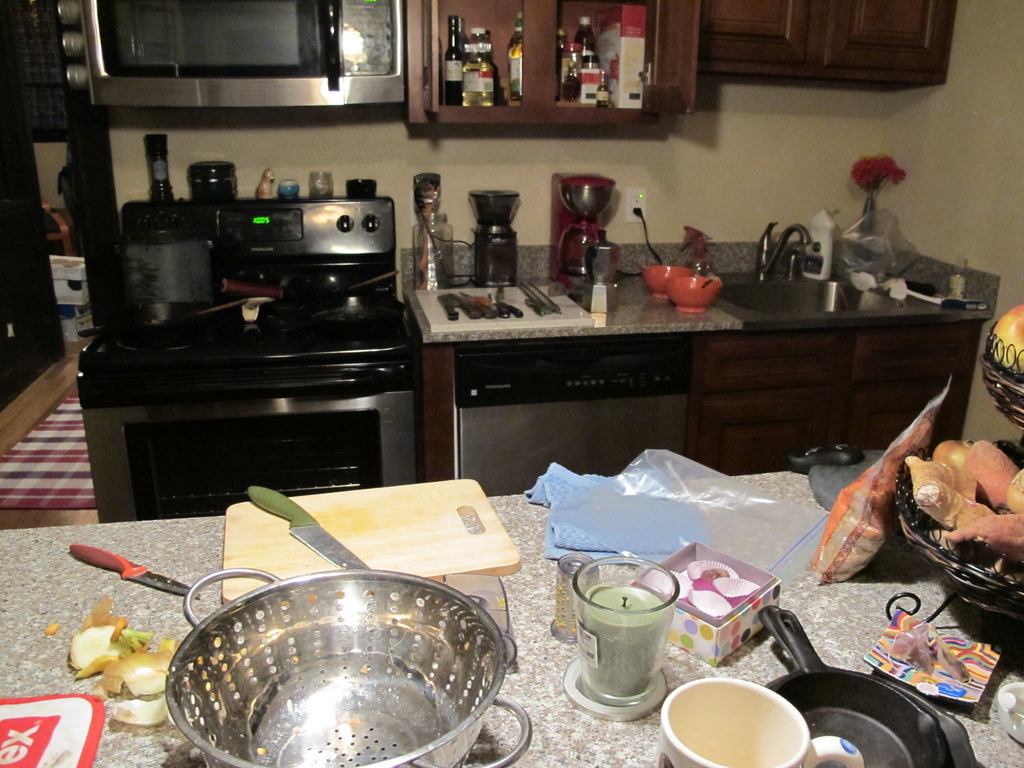The image showcases a somewhat pixelated and blurry photograph of a bustling kitchen scene. Central to the composition is an island countertop, featuring a silver metal colander, a cutting board with two knives, and remnants of a chopped onion. Nearby, an unlit candle and an open box of chocolates add a touch of warmth. To the right, a small frying pan, a mug, and a bowl containing what appears to be ginger root are visible, although the contents are not entirely clear.

In the background, the stovetop and oven anchor the view, flanked by another cutting board equipped with additional knives, located next to a coffee machine. On the far right, near the sink, two orange bowls stand out, and an upper corner of the counter displays a vase filled with vibrant flowers. Above the stove, a microwave and a cabinet stocked with various cooking oils complete the culinary tableau, adding layers of functionality and character to this domestic space.